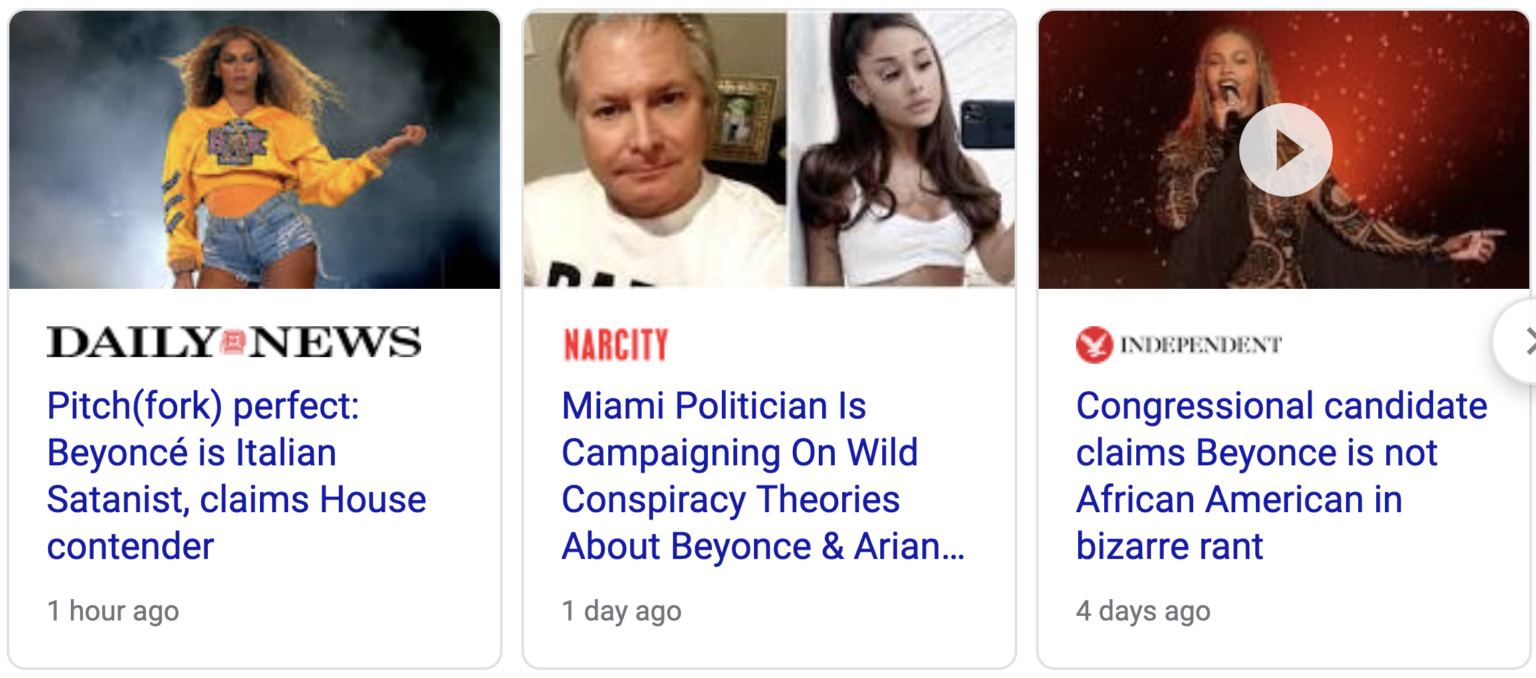This image is a screenshot of a news feed interface, displaying three distinct news articles related to Beyonce. Each article is presented within its own bordered text box, indicating that the user likely searched for "Beyonce" to generate these results.

1. The first article, sourced from **Daily News**, features a headline in bold blue ink that reads, *“Pitchfork Perfect: Beyonce’s Italian Satanist Claims House Contender”*. This headline sits above an image of Beyonce, and the article was published just one hour ago. 

2. In the middle, an article from **NARCity** is displayed with its logo in red lettering, while the title itself is in blue: *“Miami Politician is Campaigning on Wild Conspiracy Theories about Beyonce and Ariana...”*. This article, published a day ago, includes an image featuring a Miami politician alongside a side-by-side of Ariana Grande.

3. The third article, from **The Independent**, showcases their name in black text. This piece prominently features a video thumbnail of Beyonce with a play button overlay. The headline reads in blue, *“Congressional Candidate Claims Beyonce is Not African-American in Bizarre Rant”*. This news item was posted four days ago and includes a partially cut-off arrow, suggesting the option to view more articles.

The interface has a clean, organized look with gray borders separating each text box and the publication time in matching gray text. The logos of the respective news outlets are clearly displayed next to each article, contributing to the tidy and informative layout.